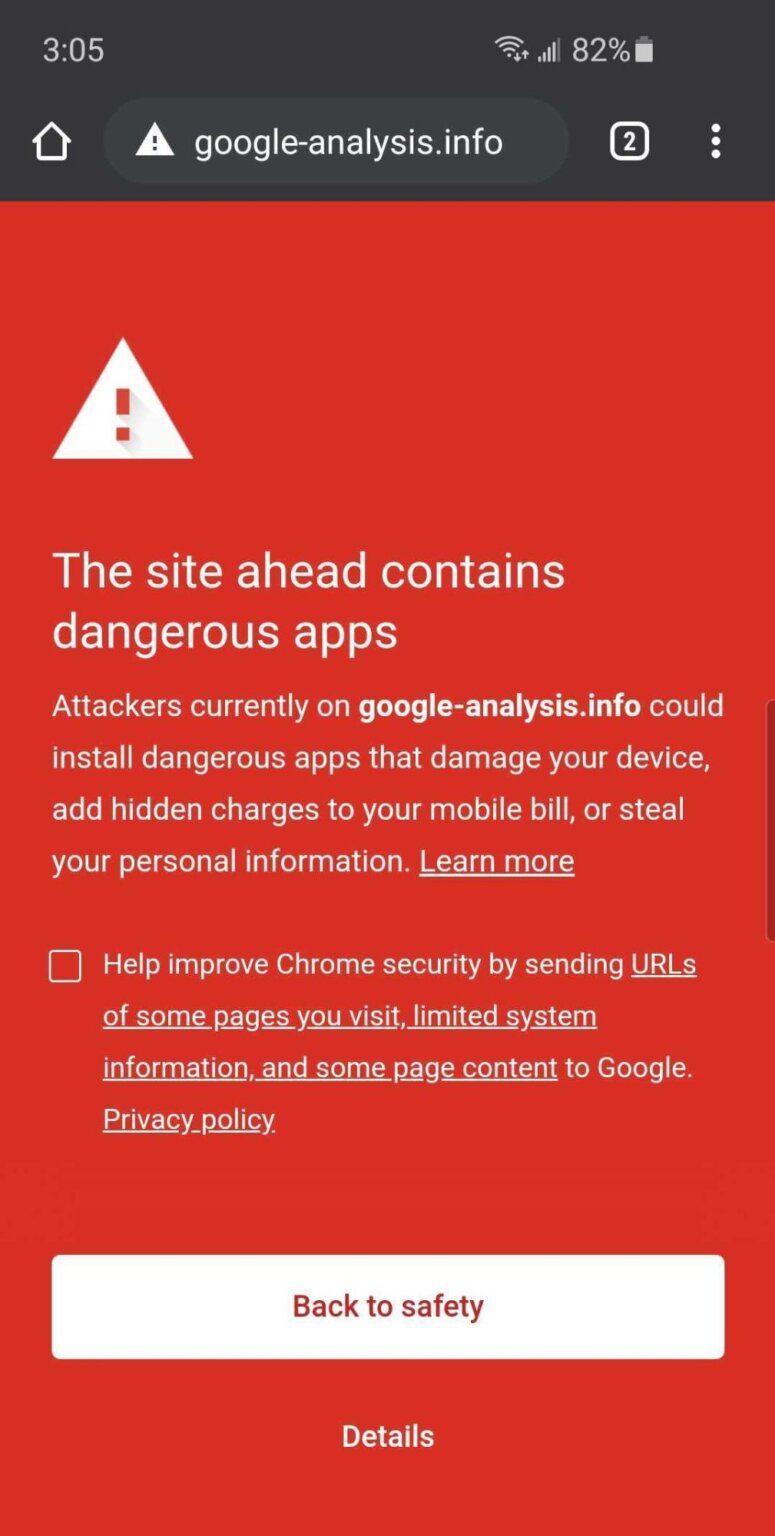A screenshot from a smartphone depicts the following details: At the top, there is a black border displaying the time as 3:05, with the device showing 4 out of 5 signal bars and 82% battery life. Below this, a home icon appears to the left, accompanied by a URL box containing a white triangle with an exclamation mark, and the address "Google-Analysis.info". To the right of the URL box, there is a small icon with the number "2" and a vertical ellipsis next to it.

Below this section, the screen turns red with a prominent white triangle containing an exclamation mark. A warning message in white text alerts the user: "The site ahead contains dangerous apps. Attackers currently on Google-Analysis.info could install dangerous apps to damage your device, add hidden charges to your mobile bill, or steal your personal information." A "Learn More" hyperlink is provided underneath the warning text.

Additionally, there is an unchecked checkbox accompanied by the statement: "Help improve Chrome security by sending URLs of some pages you visit, limited system information, and some page content to Google Privacy Policy."